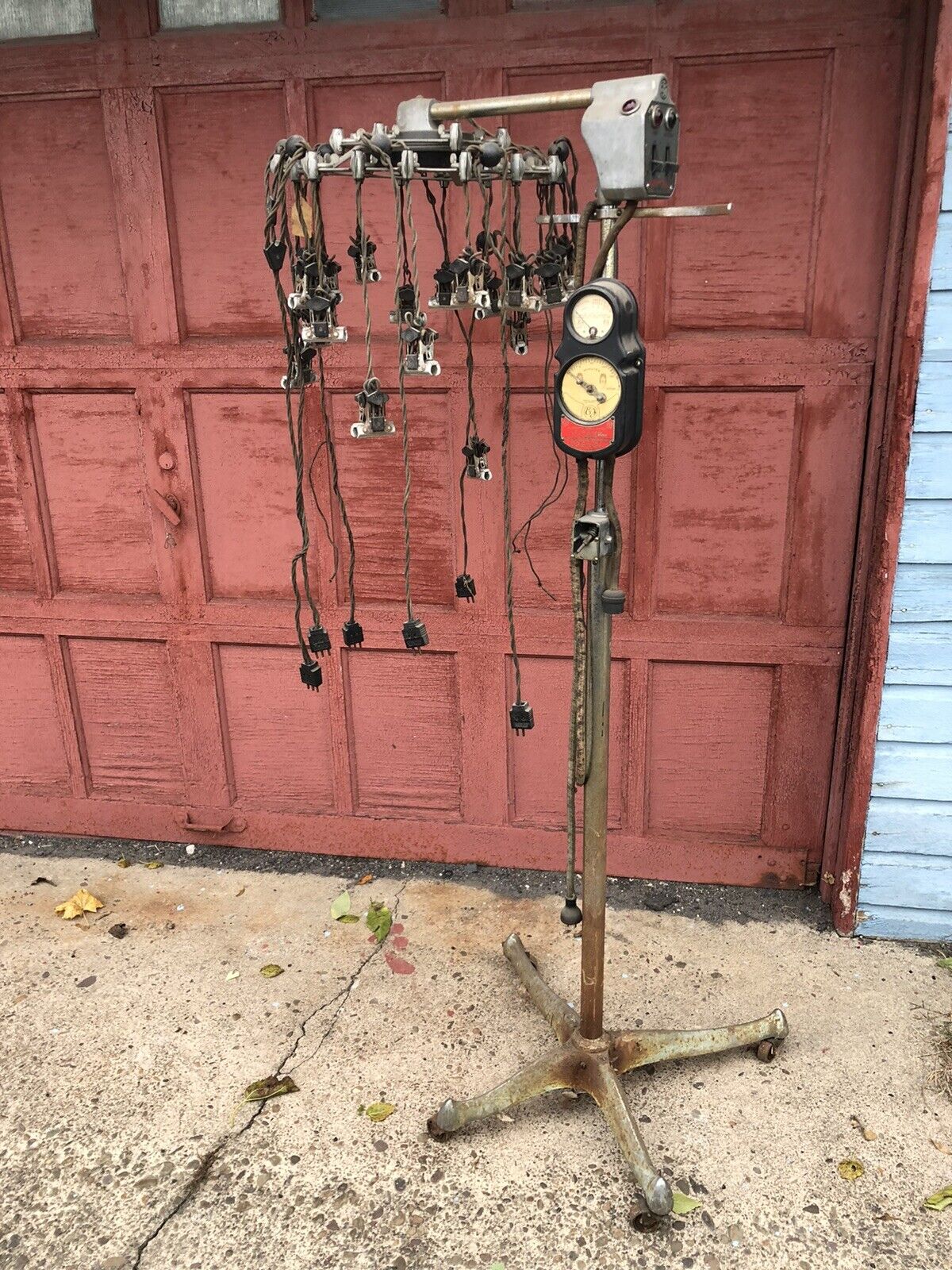The photograph captures an eerily deteriorated exterior of a garage, showcasing the weather-worn textures of both the garage door and the surrounding elements. The garage door, painted in a deep, faded red, reveals significant deterioration with wood delaminating and paint sloughing off. A small wedge of the house's clapboard siding, painted in a peeling light blue, is visible to the side, adding to the overall aged feel of the scene. The cracked and dirty concrete driveway leads up to this garage, enhancing the image's sense of neglect.

Central to the image is an unusual vintage device that resembles an old-fashioned, hospital-style rolling stand, complete with a four-wheeled metal base. The stand features a long shaft leading up to a series of dangling wires and plugs, suggesting old heating elements possibly from a vintage hair dryer. The shaft also sports what looks like a meter, possibly for voltage regulation, creating a complex and somewhat disconcerting focal point amidst the dilapidated surroundings. This strange contraption, framed against the decrepit garage door and cracked driveway, instills the scene with a haunting, almost forgotten aura.